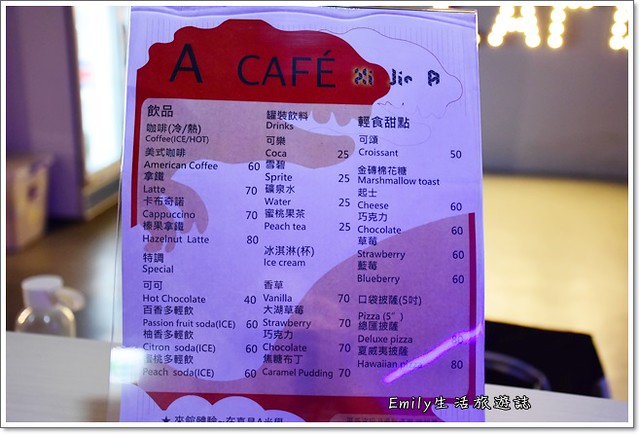This landscape-style image captures a café menu situated at the center of the frame. The background features a blurred, light brown wooden floor and a gray wall adorned with yellow LED lights, with only the letters 'A' and 'T' discernible. To the left, a blurred restaurant-style fridge is visible. 

The menu itself is vibrant with a red border and two squiggly designs placed at the top left and bottom right corners. It features both English and Asian writing, with the English descriptions listed vertically in black font. A faded white square serves as a background for the textual elements. 

The menu items include:

- Coffee (Ice or Hot): 
  - American Coffee: 60 
  - Latte: 70 
  - Cappuccino: 70 
  - Hazelnut Latte: 80 

- Specialty Drinks: 
  - Special Hot Chocolate: 40 
  - Passion Fruit Soda (Ice): 60 
  - Citron Soda (Ice): 60 
  - Peach Soda (Ice): 60 

- Cold Drinks: 
  - Coca-Cola: 25 
  - Sprite: 25 
  - Water: 25 
  - Peachy: 25 

- Ice Cream: 
  - Vanilla: 75 
  - Strawberry: 70 
  - Chocolate: 70 
  - Caramel Pudding: 70 

- Baked Goods: 
  - Croissant: 50 
  - Marshmallow Toast: 
    - Cheese: 60 
    - Chocolate: 60 
    - Strawberry: 60 
    - Blueberry: 60 

- Pizzas (5-inch): 
  - Deluxe Pizza: 80 
  - Hawaiian Pizza: 80 

At the bottom, the word "Emily" is displayed in white font, accompanied by five Asian symbols. The meticulous detailing of the menu items combined with the cozy ambiance of the café setting offers a glimpse into a quaint and inviting dining experience.